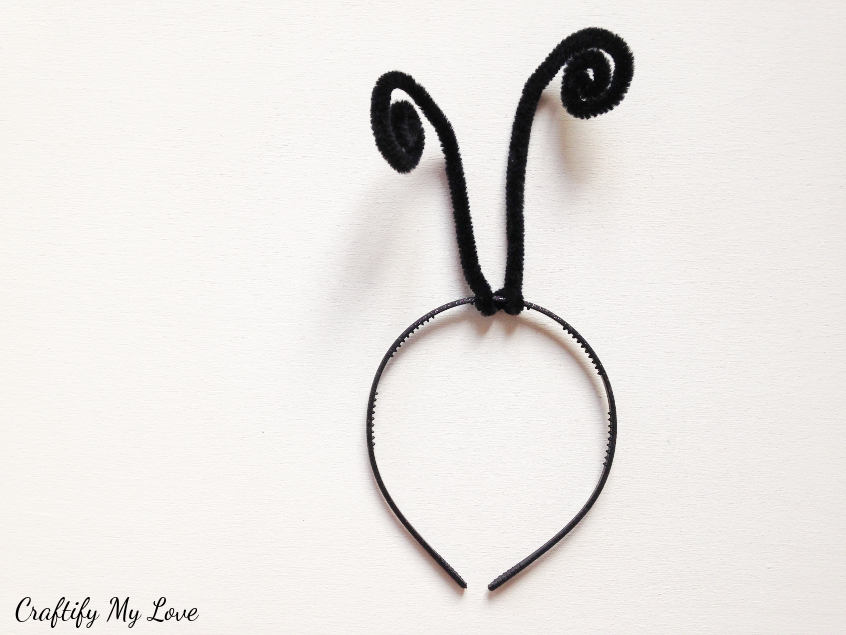The image is a color photograph with a slight landscape orientation, depicted with a subtly textured, light gray background reminiscent of paper. In the bottom left corner, "Craftify my love" is inscribed in small, black cursive lettering. Dominating the center of the photo is a thin, black plastic headband featuring small interior teeth to keep hair in place. Attached to the top of the headband are thick black pipe cleaners, styled into two whimsical, fuzzy antennae with curled ends. The headband itself is displayed in a circular shape, opening at the bottom center of the image, all captured in a realistic, product photography style.